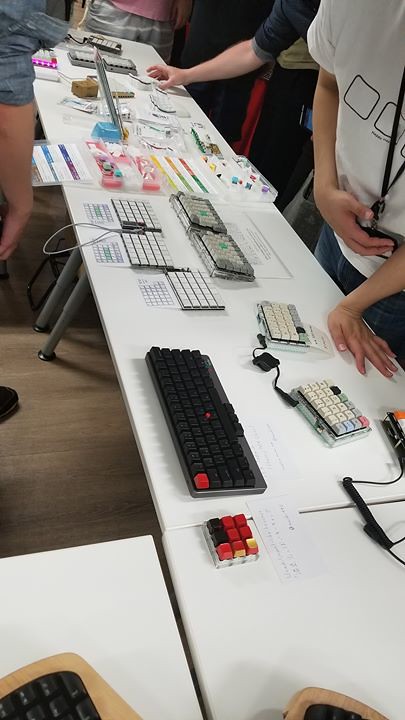The image is an indoor photograph showcasing a variety of computer keyboards arranged on a large, white rectangular table that extends from the bottom right to the top left of the picture. The table is supported by gray legs, and the scene unfolds on a wooden floor. A diverse collection of keyboards adorns the length of the table, each varying in size and color combinations. There is a black keyboard with a single red key, several smaller white keyboards with attached wires, and others featuring a mix of colors such as green, black, pink, and blue. Among them, some keyboards are flat while others are raised, and there is also a DIY craft box with rainbow colors present on the table.

In the upper right-hand corner of the image, we observe the arms of two Caucasian individuals. One person reaches down to touch the table, while the other rests a hand on it with their other arm folded in front. Surrounding this vibrant display are possibly four people, whose heads are not visible in the photograph. Notable pieces of attire include someone in a rolled-up blue button-up shirt, another person in a pink shirt paired with a gray and white striped skirt, a person in a black rolled-up dress shirt, and a woman sporting a white t-shirt with square outlines alongside jeans. Besides the multitude of keyboards, there are various elements and accessories related to keyboards scattered throughout the table, contributing to the detailed and engaging scene.